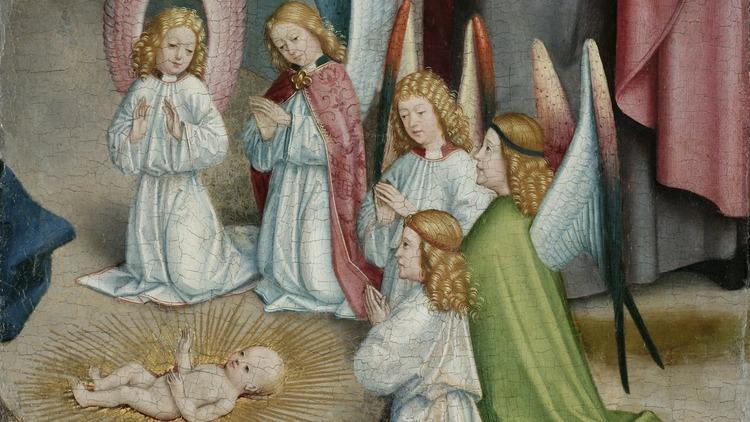The image depicts a central baby, likely symbolizing Jesus in a manger, lying on a blanket and surrounded by golden rays that resemble straw arranged in a sun-like pattern. The baby appears Caucasian with striking black eyes. Surrounding the infant are five young women, possibly angels, dressed predominantly in white robes, with some wearing red or gray over their white attire. These women, characterized by their blonde hair, have their hands together in a prayerful gesture, and most are kneeling. One notable woman, older than the others, wears a distinctive green cape. The background features gray and red curtains, creating a solemn and reverent atmosphere reminiscent of an old-fashioned religious painting from the Renaissance period.